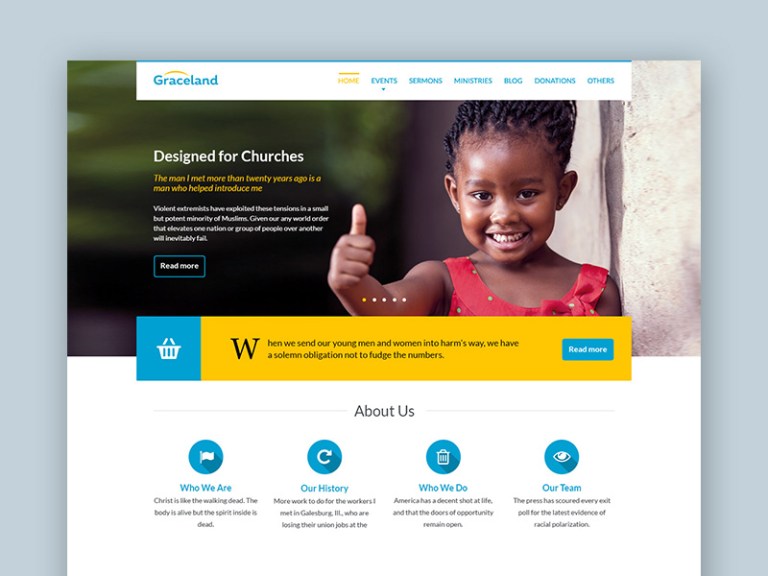Certainly! Here's a cleaned-up and detailed descriptive caption for the image based on your description:

---

The image displays a homepage interface seemingly related to church services and community activities. Dominating the top section is the name "Gracelyn" prominently written in blue letters with a yellow symbol above it. Adjacent to this are navigational tabs labeled "Home" in yellow letters, followed by "Events," "Sermons," "Ministries," "Blogs," and "Donations."

Below this header, there is a photograph of a young Black girl looking cheerful and giving a thumbs-up gesture. She is wearing a sleeveless red dress, which appears to be a light and summery attire.

To the right of the girl, there's a white text that says "Designed for Churches." Beneath this, there is a yellow-highlighted quote reading: "The man I met more than 20 years ago is the man who helped introduce me," next to contextual information in yellow about violent extremism and global tension. An incomplete statement about a world order follows, with a "Read More" option at the end.

Further down, there is a blue and yellow banner. On the left side of the banner, there is a graphic of a white basket. The yellow portion contains the message: "When we send our young men and women into harm's way, we have a solemn obligation not to fudge the numbers," followed by another "Read More" option.

The section below features various tabs, beginning with "About Us." The immediate subheading under it is "Who We Are," paired with a quote: "Christ is like the walking dead, the body's alive but the spirit inside is dead," and a loading spinner icon. Next is "Our History," which mentions workers in Galesburg, Illinois, losing their union jobs. Following this is "What We Do," stating, "America has a decent shot at life, that the doors of opportunity remain open." The final tab is "Our Team," which includes a reference to media analysis of radical polarization. Notably, this section also has an icon resembling a small garbage can.

Overall, the text content appears somewhat disjointed and may contain references that are unclear or out of context, potentially hinting at the creator’s non-native English proficiency. The overarching theme seems to center around church services and community support.